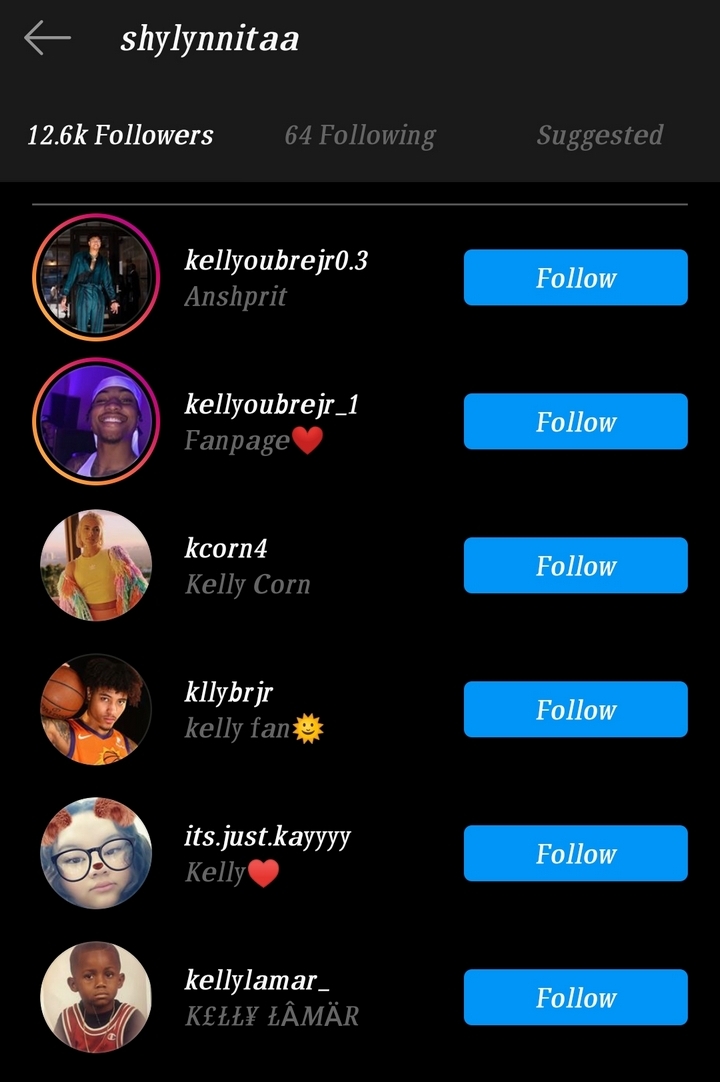The image captures a screenshot from Instagram showcasing the followers list of the user "ShyLanita". The interface features a black background with a gray arrow in the top left corner, allowing navigation back to the main page. Highlighted in white at the top are three key metrics: "12.6k followers," "64 following" (grayed out), and "suggested" (also grayed out). The followers section is currently selected.

Beneath these metrics, the screen lists six Instagram users who follow "ShyLanita." Each follower is presented with a circular profile picture on the left, their username in white next to it, and a brief description below each name. While some descriptions identify as fan pages, others are simply names.

On the right side of each follower's entry, there is a prominent blue button labeled "Follow" in white text, available for "ShyLanita" to follow these users back.